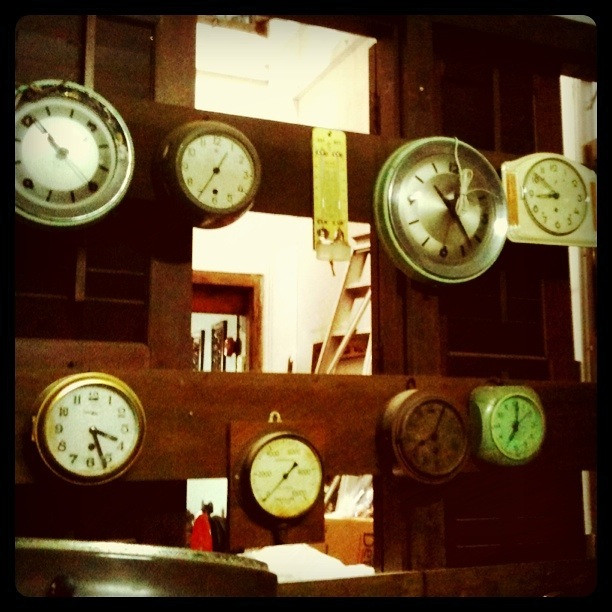This square, vintage-looking photograph, framed in black, exudes an aged charm with its grainy texture and muted color palette. The image, reminiscent of an early 20th-century capture, features a rustic wooden wall with sections that reveal a room beyond. Dominating the scene are two prominent wooden slats that span the width of the wall, from which an eclectic collection of round clocks dangle. Each clock, varying in size and style, adds to the nostalgic ambiance. Some clocks boast complete numerical dials, while others display only the cardinal points of 12, 3, 6, and 9. The frames differ in finish, ranging from opulent gold to sleek silver, enhancing the diversity within the uniformity. The overall effect is a visually striking array of timepieces, each with a unique history, collectively evoking a sense of timelessness and antiquity.